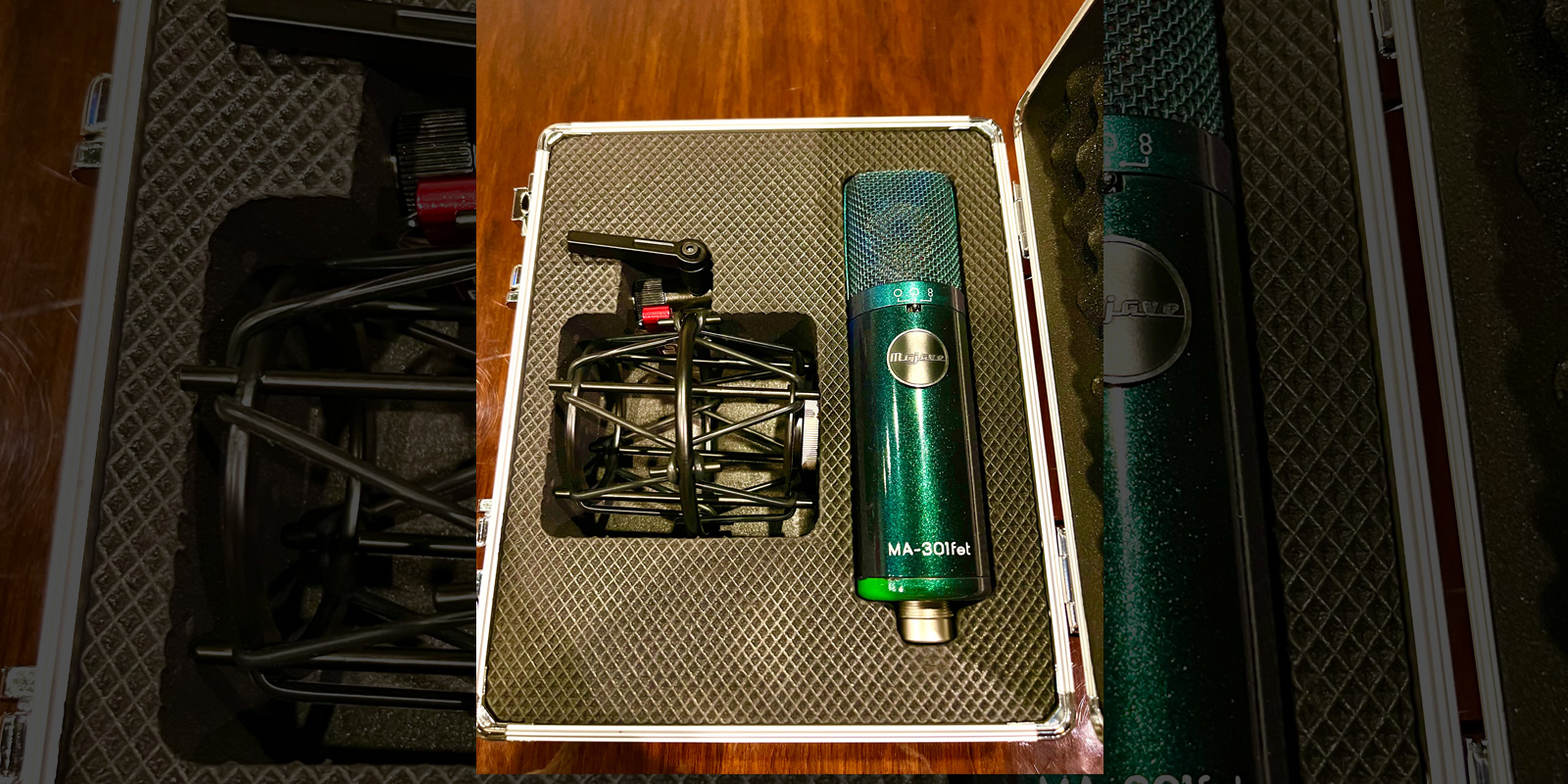This detailed photograph captures an indoor scene featuring an open case with a wooden floor as the backdrop. The case, resting likely on a wooden table, reveals a meticulously arranged set of audio equipment. At the forefront, a green microphone, labeled "MA 301 FET" with a distinctive golden logo that appears to read "ME JAVE," dominates the right compartment. The microphone, potentially custom-painted, is surrounded by compartments designed to securely hold its components. On the left, other microphone parts, including a filter and a base, are snugly placed within the case's honeycomb-shaped padding. The interior lid of the case is lined with eggshell foam, providing additional cushioning for the equipment. The detailed layout and careful arrangement suggest a professional setup, with the wooden flooring enhancing the overall presentation.